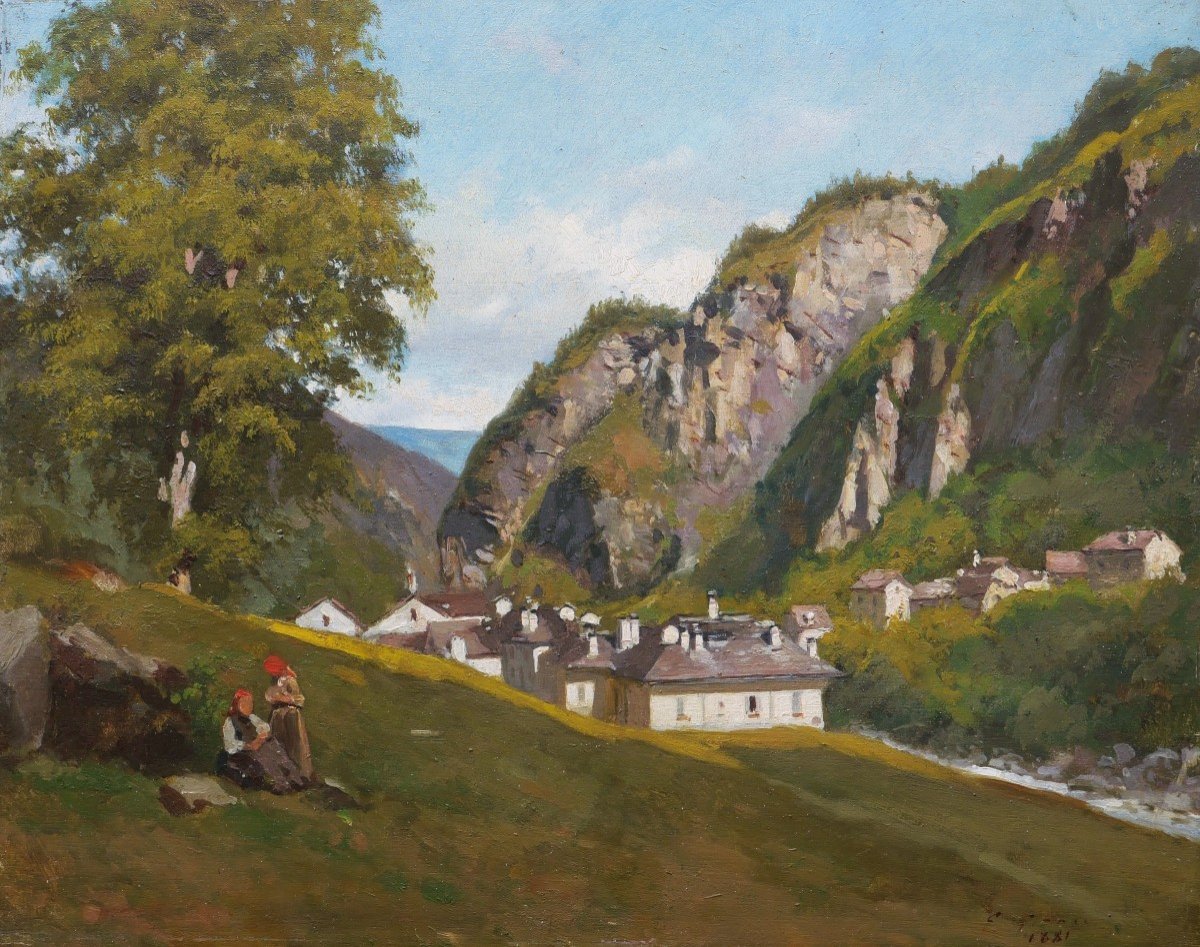This is a detailed color painting of a serene countryside scene in a landscape orientation. The background features a light blue sky dotted with white clouds. On the right side of the image, a rocky cliff or canyon covered in green vegetation extends to the top right corner. This jagged cliff slopes downwards to meet a small village nestled at the bottom of the valley, with a creek or brook running through the center. The village is comprised of white houses with brown rooftops, arranged in two clusters: some are situated directly below the cliff and others lie on the opposite side of the ravine.

On the left side of the painting, a gentle hillside slopes downwards, adorned with light green foliage and a prominent tall tree that reaches the top left of the image. In the bottom left corner, there are two figures, likely ladies, identified by their red headgear which resembles bandanas. One is seated beside a large grayish brown boulder, and the other stands next to her, both appearing to be enjoying a restful moment. This idyllic scene, complete with a hillside, a picturesque village with quaint houses, and elements of natural beauty, evokes a sense of tranquility and harmony with nature.